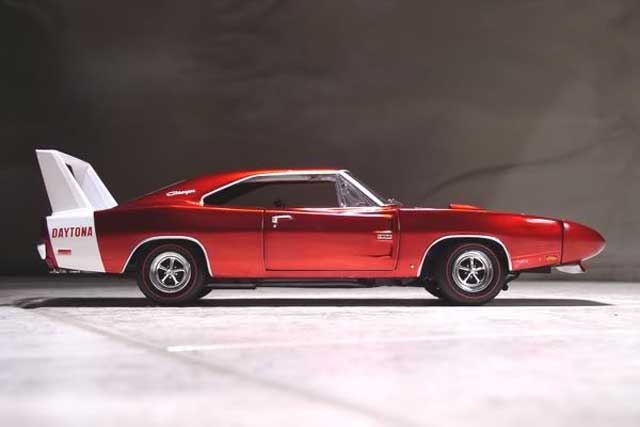The image showcases a sleek, shiny red sports car with a white tail fin that wraps around the back, emblazoned with the word "Daytona" in red text. The car is positioned on a gray surface that resembles tile flooring, hinting that it might be a toy car. From the side view of the passenger side, the two-door car features chrome handles, a large and thin front end, and black tires with chrome centers. The car is well-illuminated from a light source above, casting clear shadows underneath, and the dark gray to almost black background contrasts sharply with the light gray floor. The open window adds to the detailed and reflective elements of the car's surface, further enhancing its realistic appearance.